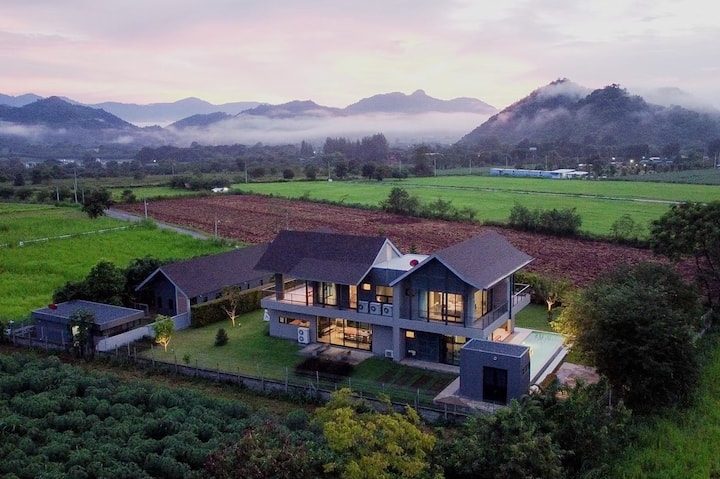This image is an aerial view of a sprawling modern property set against a lush landscape. In the foreground, a large, two-story house dominates with a brown roof and several glass doors and windows, giving it an open and contemporary look. The house features multiple balconies, a spacious deck, and a patio area. Adjacent to the main house is a standalone structure that appears to function as either a garage, greenhouse, or another work building. A smaller, gray building with a flat roof is also part of the property, forming a complex of three distinct structures.

Surrounding the house, a fence with a wall encircles the immediate area, separating the manicured grounds from a forested region. The yard boasts a pool, and warm light emanates from inside the house, although it is daytime. The sky is a blend of white, pink, and light blue hues, with some clouds and fog beginning to settle in.

Beyond the property, the landscape features a mix of green fields and a large, recently plowed brown field in the middle of the greenery. Light trees sprinkle around these fields. In the distance, a line of trees marks the horizon, backed by a misty mountain range, which adds to the serene and picturesque setting.